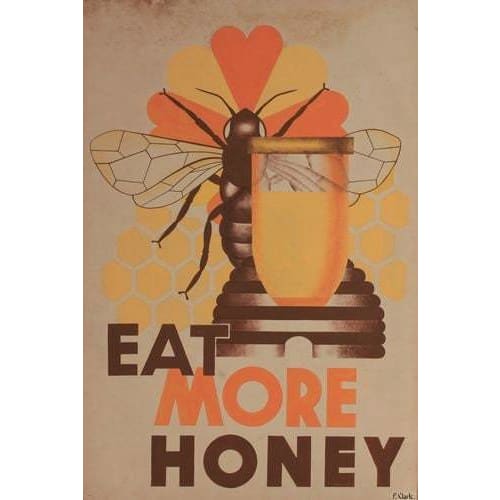This detailed poster advertisement, reminiscent of the 1950s and 60s art style, promotes the consumption of honey with its bold text, "EAT MORE HONEY," written in all capital letters. The word "eat" and "honey" are in black, while "more" stands out in red. The background of the poster is a slightly faded beige, indicative of its vintage nature. At the center top, a honeybee with clearly detailed beige, white, and yellow wings and a distinctly black abdomen and legs is prominently displayed. The bee is perched on an alternating orange and yellow flower, with a golden honeycomb pattern in the background. Positioned in front of the bee is a clear jar of honey with a bronze lid, partially filled with golden-yellow honey. Additionally, a honey stick is layered between the bee and the jar, adding another classic touch to this nostalgic and richly illustrated advertisement.